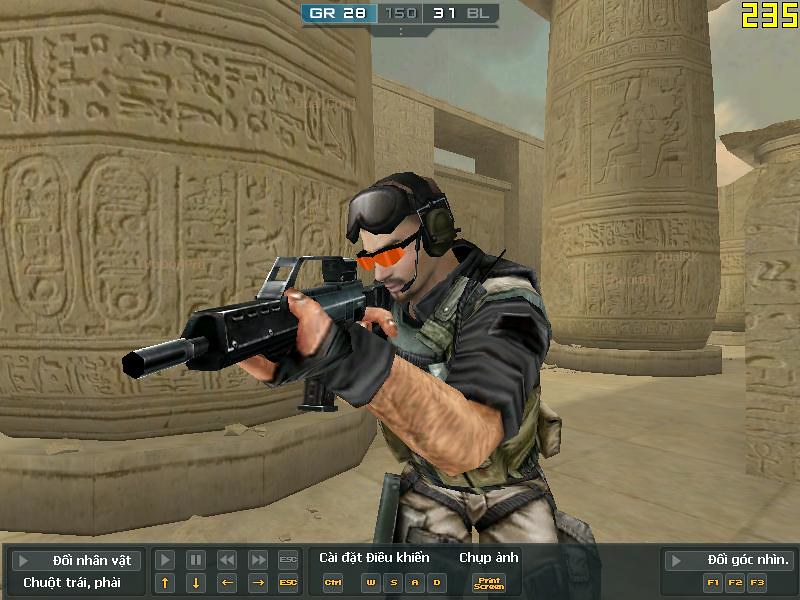In this slightly horizontally rectangular screenshot from a video game, the scene is set against a backdrop reminiscent of ancient Greece or Egypt, with large tan structures and elaborately carved columns evoking a historical ambiance. At the top center of the screen, statistical data is displayed, while a banner at the bottom—written in a non-English language—features various selectable buttons. Dominating the center of the image is a heavily-armored soldier, his body facing the camera but turning slightly to his left to aim a rifle downward. He is clad in military attire, including a dark black shirt with sleeves rolled up to reveal his hairy arms. The soldier is equipped with a helmet, headphones, and protective goggles perched on his forehead, along with orange-tinted glasses shielding his eyes. His intensely focused posture and detailed gear contribute to the immersive and dynamic nature of the game.